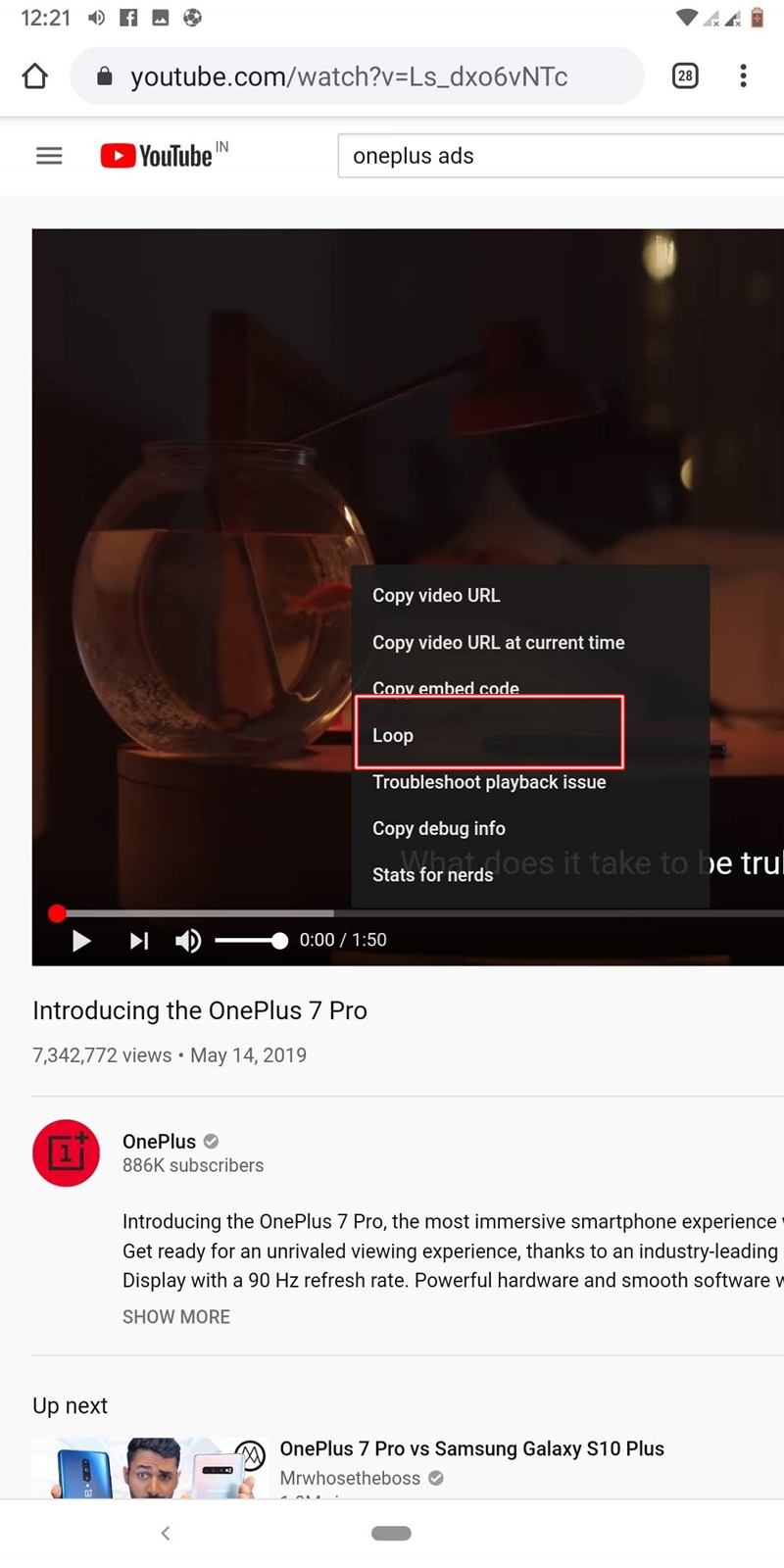The image is a detailed screenshot of a YouTube web page interface. At the top, the time is displayed in the left-hand corner along with several icons, including a sound icon, a Facebook icon, a calendar icon, and another small, unreadable icon. On the far right, additional icons are visible: a Wi-Fi icon, a signal icon, and possibly a battery icon. Below this row, the home icon and a search bar can be seen.

The URL displayed in the address bar reads "youtube.com/watch?v=LS_DXO6VNTC," with a lock icon indicating it's a secure connection. To the right of the search bar, there's a square icon with the number "28" and a menu icon represented by three vertical dots. Below these, there's another menu icon consisting of three horizontal bars stacked vertically.

Adjacent to the address bar, the YouTube logo appears as a red play button followed by the word "YouTube" in capitalized letters. The search bar also mentions "1+ ads."

Beneath the search bar is a picture image section that presents several options, including "Copy video URL," "Copy video URL at current time," and others. There is a "Loop" option within a black rectangular box outlined in red.

Further down, the video's play time and play buttons are visible. The main content of the page features a video titled "Introducing the OnePlus 7 Pro," with an impressive view count of "7,342,772 views" and a publication date of May 14, 2019. The OnePlus logo, a red circle with a white square inside containing the number "2" and the text "OnePlus," is displayed beneath this information.